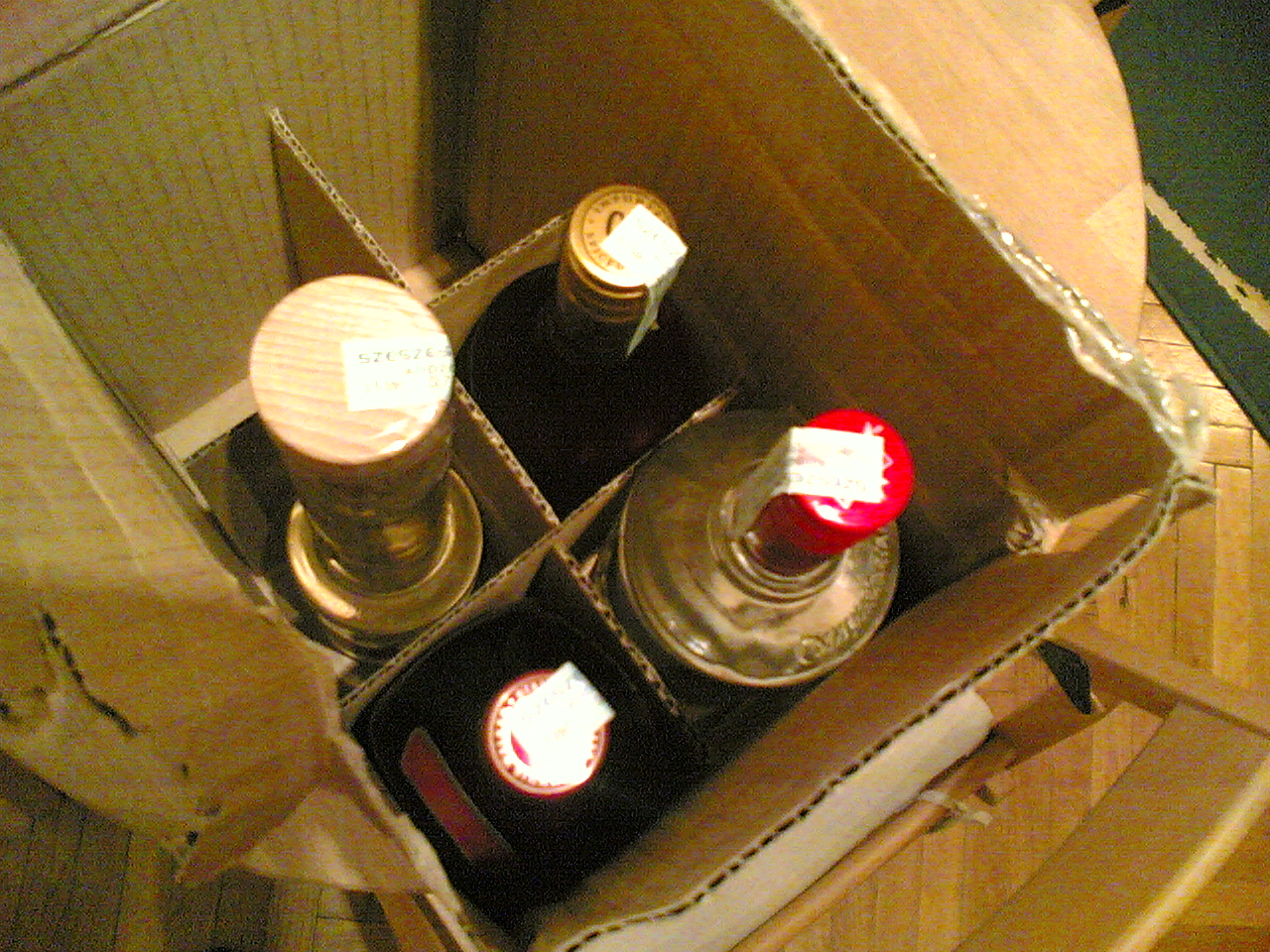This top-down photograph captures a brown cardboard box with six compartments, situated on a light wooden table. Four compartments are occupied by various bottles, while two remain empty. The contents include:

- A light brownish bottle with a cork, potentially olive oil.
- A brown bottle, possibly liquor or brandy, with a golden twist cap.
- A transparent bottle featuring a vivid red twist cap, likely vodka.
- A square dark brown bottle, adorned with a red cap and rectangular label with golden letters.

All bottles are sealed with paper stickers running from the bottle neck to the cap, indicating they are unopened. The box is taped around the edges and placed on a table, which matches the light wooden parquet floor below. In the background, a green rug is partially visible. A chair is pushed under the table, completing the setting.